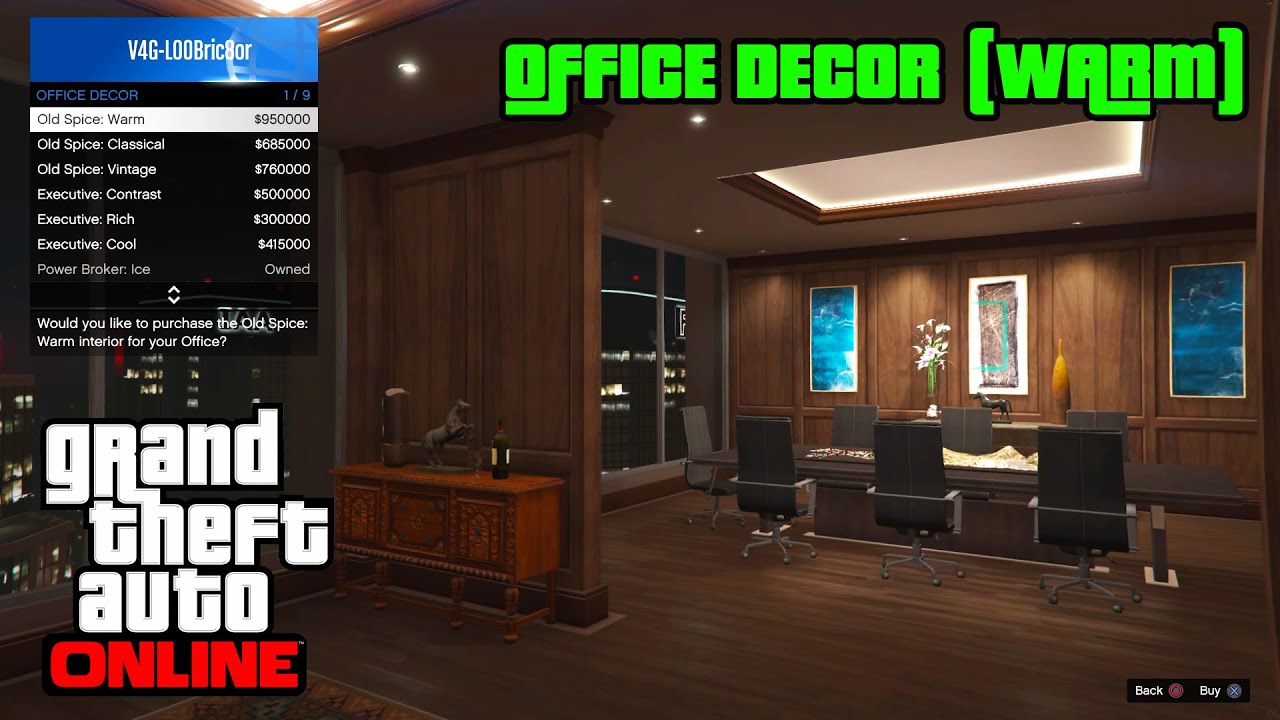This image is a detailed screenshot from the video game Grand Theft Auto Online. The photo prominently displays the game's trademark font in the lower left corner, labeling it as "Grand Theft Auto Online." At the top of the image, vibrant green text reads "Office Decor" with "Warm" in parentheses, indicating the theme of the in-game office customization option showcased in the screenshot.

The scene depicts a large, open office space decorated with wooden paneling and three distinct paintings on the wall. The centerpiece of the room is a long, dark wooden conference table surrounded by seven black, rolling chairs. To the left, there is a menu interface offering different office decor options at various prices, ranging from $950,000 to $41,000, allowing players to customize their in-game environment.

The office features large steel-framed windows that open up to an urban skyline, suggesting the office is situated high in a multi-story building. Additionally, a closed shelf and other furnishings are visible, enhancing the office's detailed and immersive design. The overall aesthetic, complete with dark brown accents and high-end decor options, provides a sophisticated and customizable virtual workspace experience.